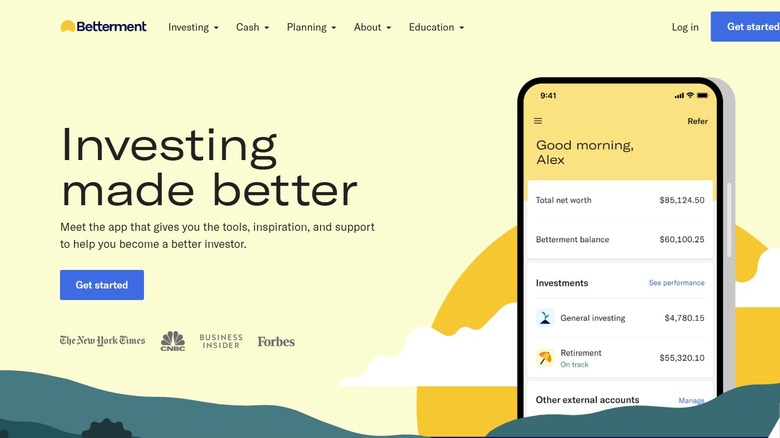This is a cropped screenshot of the home page of the Betterment website, featuring a light yellow background with minimalist graphics. At the bottom of the page, there is a blue silhouette of hills and the top of a tree on the bottom left, depicted as a silhouette. To the right of the tree, there are abstract yellow paint strokes positioned behind an image of an iPhone. The iPhone displays the Betterment app interface on its screen. 

On the left side of the page, bold black letters proclaim, "Investing made better." Beneath this, in smaller black text, it reads, "Meet the app that gives you the tools, inspiration, and support to help you become a better investor." Further down, there is a prominent blue bar with white text that says "Get Started."

At the very bottom of the screenshot, logos for the New York Times, Business Insider, and Forbes are visible. At the top left of the page, next to the Betterment logo, are navigational categories labeled Investing, Cash, Planning, About, and Education, each with drop-down menus. On the far right, there are options to log in or get started, with the "Get Started" option appearing in a partially cropped blue rectangular bar.